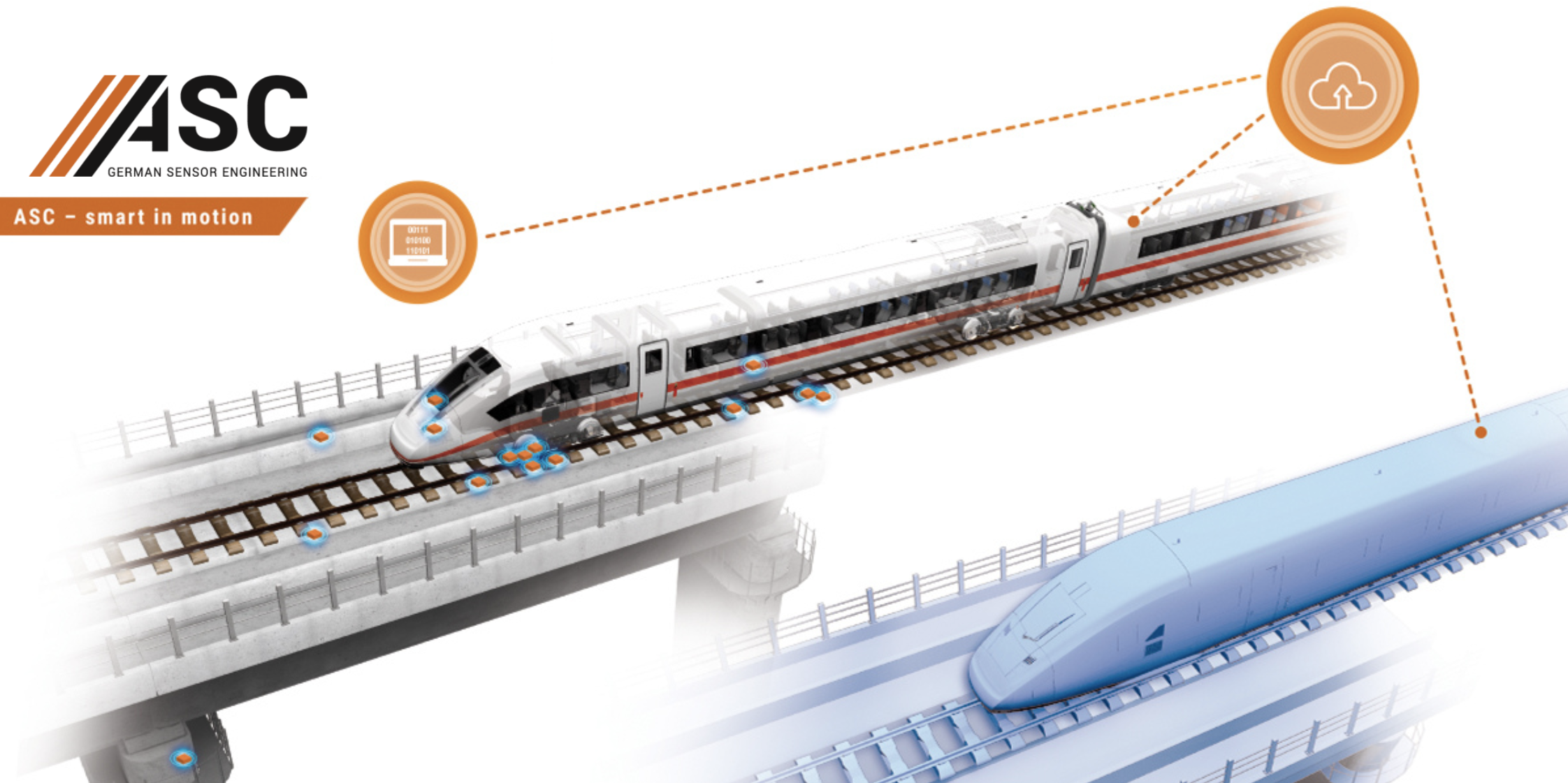This infographic illustrates ASC's German Sensor Engineering for high-speed trains, titled "ASC - Smart in Motion." Dominating the image are two parallel sets of elevated train tracks, each with a distinct train model. The train on the left track is completely blue with a sleek and advanced appearance, while the train on the right track is white with black and red stripes, featuring visible windows and doors, and a transparent design that reveals the seat arrangement inside.

In the top left corner, an ASC logo is displayed, featuring black text with orange accents on the letter "A." At the bottom, an orange ribbon bears the text "ASC - Smart in Motion" in white letters. Key visual elements include two orange circles: one on the left side with a computer symbol, and another on the right side with a cloud and an upward-pointing arrow. A dotted line connects the computer symbol to the cloud, signifying data transmission, from which two additional dotted lines extend to each train, indicating a smart control system that connects the trains to the central computer via the cloud. This setup emphasizes the integration of advanced sensor technology and data management in optimizing train motion and performance.